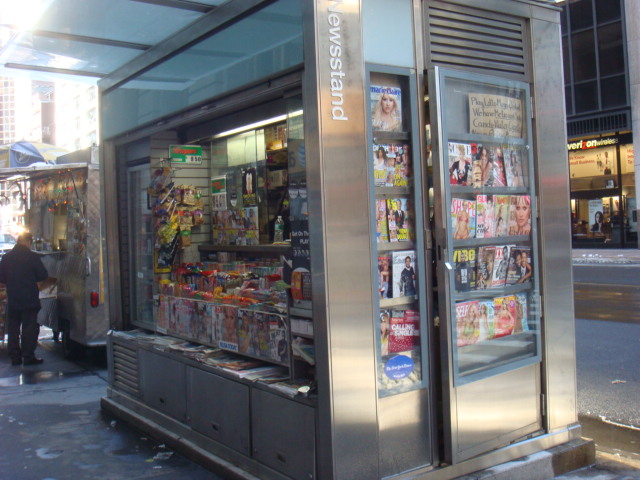This is a color photograph capturing a small, urban newsstand positioned right next to the street on the sidewalk. The rectangular kiosk is constructed of stainless steel with white lettering spelling "newsstand" on one of the metal pillars. Viewed from a diagonal angle, the image reveals shelves and display cases brimming with magazines on the exterior walls, particularly on both the left and front sides. A partially open door on the right-hand corner leads inside, where additional shelves of magazines are visible. Hanging from the walls and behind the counter are various snacks. In the background, towards the right, a street is visible along with a set of shops, including what appears to be a Verizon store. The bustling urban scene is further accentuated by another man dressed in black, seen in the background near a silver vehicle or another stand. The area appears lively with lit shop windows and multiple buildings framing the scene.